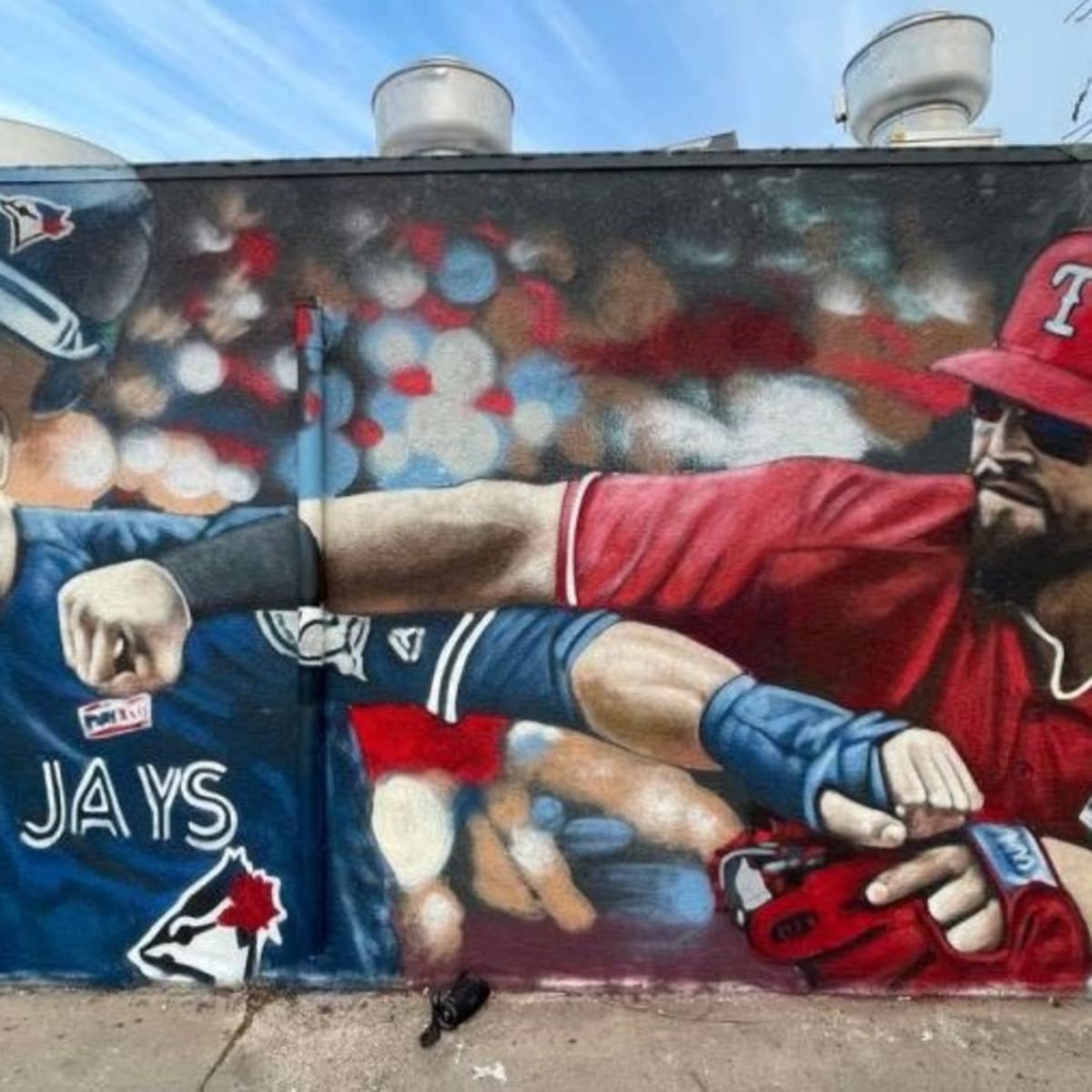The mural captures a tense and dramatic moment of a brawl between two baseball players against a backdrop of a light blue sky. The left player, clad in a Toronto Blue Jays jersey and helmet, is a white man with his helmet partially dislodging. He is swinging his left fist towards his opponent. The right player, in a red jersey with a 'T' on the cap, indicative of a Texas team, is a black man wearing a red glove, who is retaliating with his right fist. The scene unfolds on a dirty, cracked concrete sidewalk, lending a gritty realism to the painting. Behind the players, a blurred stadium roof and people add to the chaotic atmosphere, emphasizing the intensity of the fight.